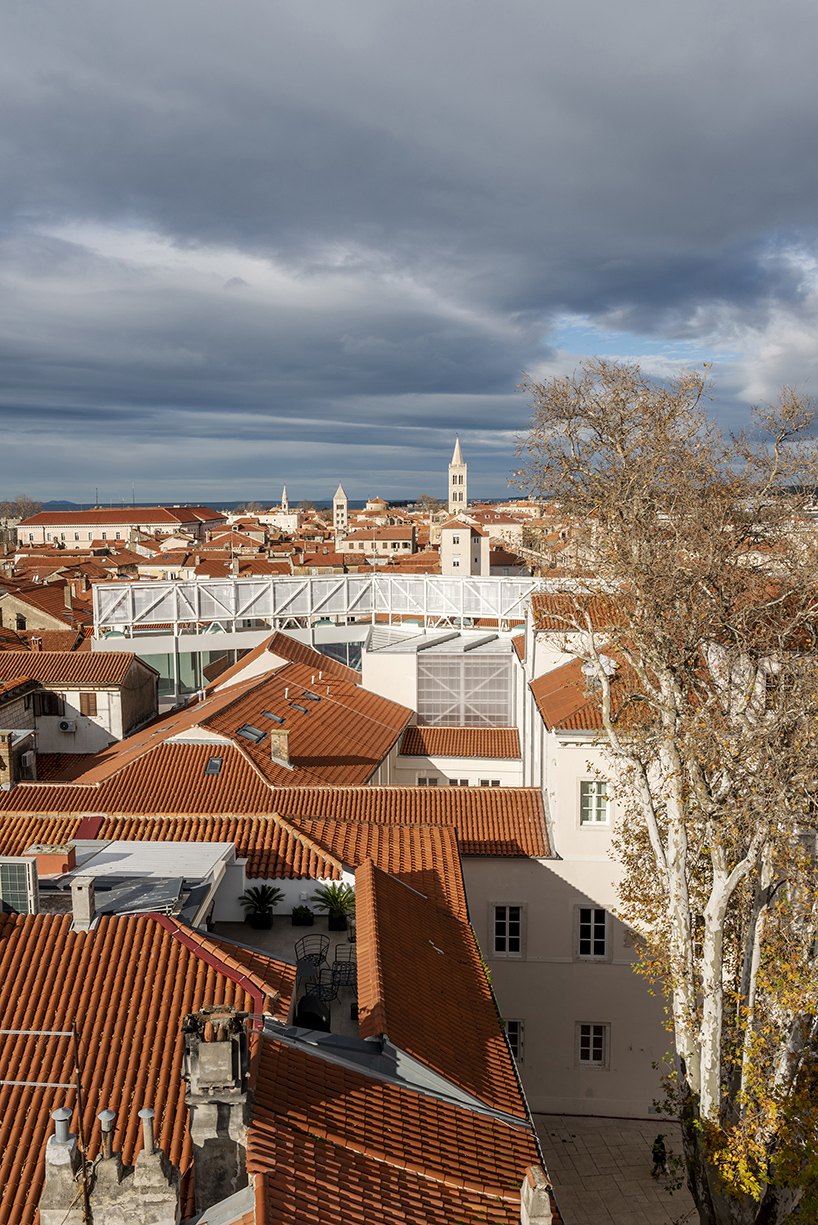This photograph captures an aerial view of a small European town on a cloudy, overcast day. The top third of the image showcases a sky filled with dark gray clouds, with a small patch of blue sky visible on the right. Dominating the right side of the photograph is a tall tree with a white trunk and rust-colored leaves. Beneath this dramatic sky, we see a landscape of cream-colored and white buildings, each featuring ornate, curved terracotta tile roofs that are rich in orange and rust hues. The town is densely packed with two to three-story homes, many of which have tall steeples and multiple chimneys. In the heart of the town, a white metal bridge stretches across the center of the photograph, adding an architectural charm. In the distance, tall church steeples rise above the horizon, hinting at historical significance. There are glimpses of water far in the background, further framing this picturesque and timeless scene.